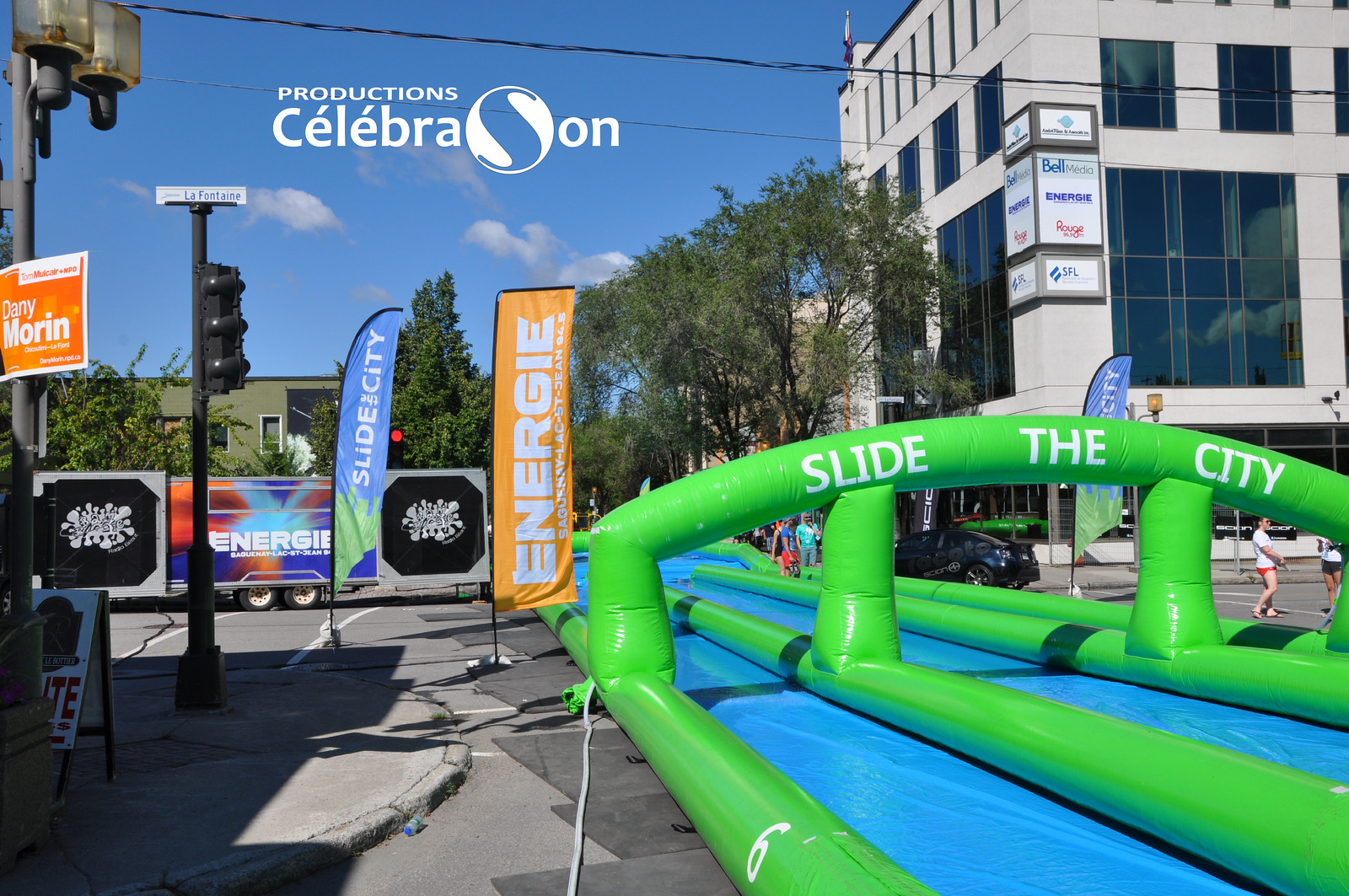The image features an oversized inflatable water slide, prominently positioned in the middle of a large city street, effectively taking up most of the roadway. This slide, branded with the words "Slide the City" at the top, is primarily blue with green inflatable supports. In the background, various advertising flags can be seen, one with white letters on a yellow background reading "Energize," and another with a blue and green background stating "Slide City." 

On the right side of the slide, a few people are visible, engaging with one another in a lively manner. Nearby, there are several trucks and vehicles parked along the streets. Dominating the right side of the frame is a significant, multi-story concrete building, approximately four or five stories high. Additional buildings and power lines are noticeable in the surroundings, along with trees that have leaves, indicating a temperate season. The sky above is clear with a few scattered clouds, suggesting the photo was captured during the daytime.